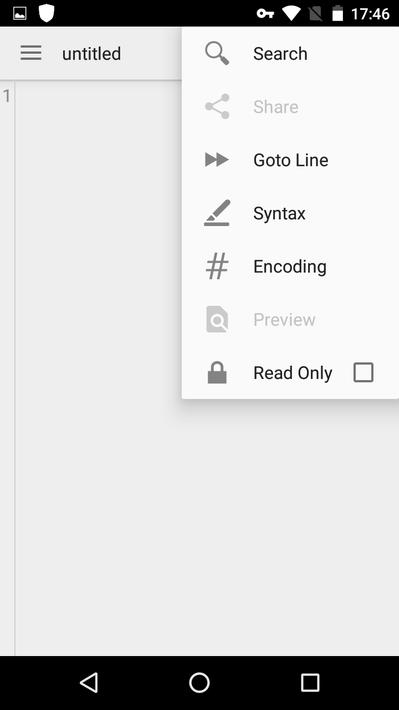This image is a detailed screenshot of a coding or text editor interface on a mobile device. In the top left corner, a gallery symbol and a shield icon are visible, indicating some form of content protection or verification. The top right corner displays several status icons: a key, a Wi-Fi symbol, a grayed-out SD card, and a battery indicator showing approximately 75% charge. The current time is 17:46.

Below the status bar, there’s a gray box labeled "Untitled" featuring three black horizontal lines. Adjacent to this, a number "1" is displayed, presumably indicating the line number. 

The interface includes a search bar and several function buttons labeled "Share," "Go to Line," "Syntax," "Encoding," "Preview," all appearing below the gray box. Except for "Share" and "Preview," which are gray, the other labels are black. Near the bottom, a black box is labeled "Read-Only," indicating that the document might be in a non-editable state.

The overall background is a solid gray while the top and bottom areas are black. The bottom bar contains three navigation icons: a white arrow, a circle, and a square. Additionally, there is a faint, skinny black line running vertically downwards on the right side of the number one, suggesting a possible cursor or delimiter within the text editor.